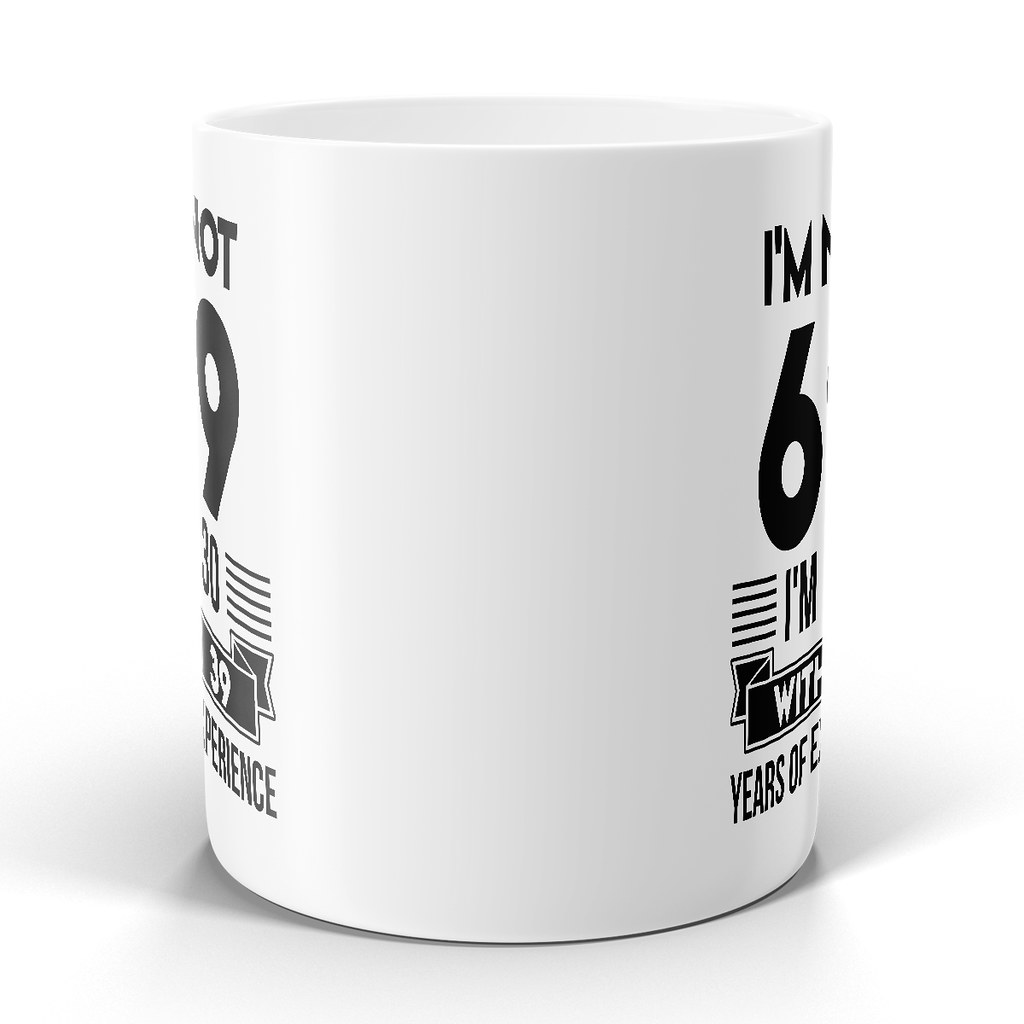In the image, there is a white mug set against a pure white background. The mug is oriented so that its handle is not visible, showing primarily the front and parts of both sides. The front of the mug is completely white, while its sides feature a distinctive black design that wraps around.

On the left side of the mug, at the top, it reads "not," followed by the number "9," then "30," and beneath them in a black strip, the number "39." At the very bottom, the end of a word "experience" is visible.

The right side of the mug shows the phrase "I'm," with a prominent "6" right below it, followed by another "I'm" positioned directly below the "6." Additionally, the number "30" appears above a black banner reading "with," followed by the phrase "39 years of experience" split across several horizontal lines. 

This design cleverly merges the words "I'm not 69, I'm 30 with 39 years of experience" in a visually segmented manner, utilizing the curvature of the mug for a playful and intricate presentation.